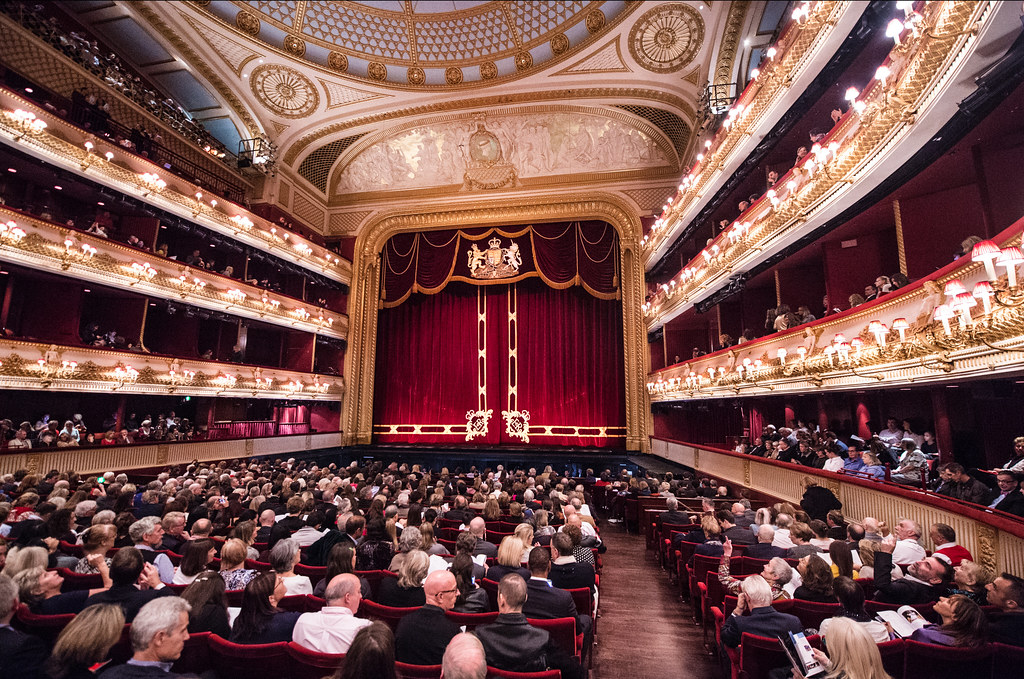This image depicts an opulent concert hall or theater with a grand atmosphere. The perspective is from an aisle, looking towards the stage, capturing details that emphasize the richness and elegance of the space. The focal point of the image is the stage, adorned with large red curtains featuring gold trim and intricate detailing. Above the stage, a gold-colored arch crowns the setup, and atop the curtain hangs an ornate fabric with a emblem showcasing two lions climbing onto a shield topped with a crown, all in gold.

The seating area is filled with people, many dressed in suits and white shirts, adding to the formal ambiance. The seats themselves are a plush red velvet. The hall is structured with multiple levels of balconies, possibly three or four tiers, each fronted with white exteriors and golden fixtures, adorned with lights. The balconies are populated with more audience members, and the highest tier offers a visible glimpse of the white ceiling also detailed with gold trim.

The flooring is brown, and the front wall of the stage area is outlined in gold and white. The overall impression of the venue highlights its grandeur and sophisticated design, filled with intricate gold accents, red velvet elements, and a well-dressed, attentive audience.